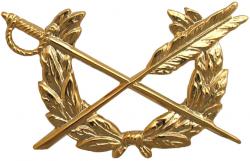The image displays an intricately designed golden insignia set against a stark white background. Central to the design is a diagonally positioned sword, with its handle in the upper left corner, extending downwards to the lower right. Crossing the sword is a golden arrow oriented from the upper right to the lower left. Surrounding the central elements is a golden laurel wreath that curves upwards, forming a U-shape with an open top, somewhat reminiscent of two upward-pointing horns. This emblematic piece, which could be a pin, pendant, or charm, features detailed and elegant craftsmanship that suggests it serves a significant symbolic or decorative purpose.